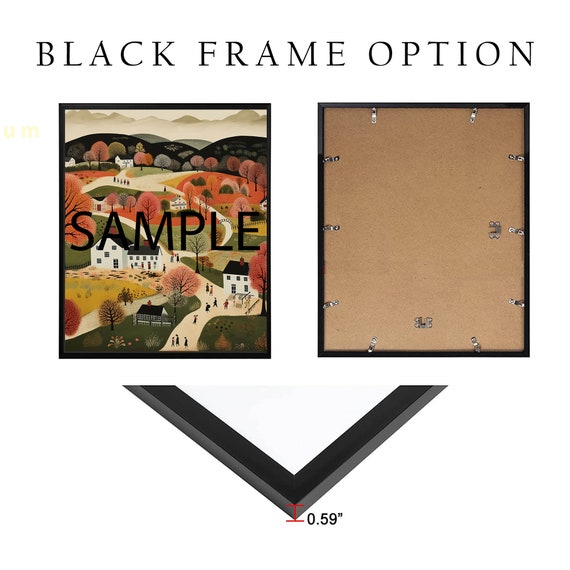The image showcases two picture frames against an all-white background under the text "BLACK FRAME OPTION" in black, capital letters. The left frame features a forward-facing view, illustrating a vibrant, multicolored town with rolling hills, trees, white houses, and tan pathways. This illustration has "SAMPLE" prominently displayed in black letters on its surface. The frame itself is thin and black. The right frame provides a rear view, displaying the brown cardboard backing secured by silver clasps and equipped with a hook for hanging. Below these frames is a close-up detail of the frame's corner, marked with the measurement ".59" indicating the frame's width.